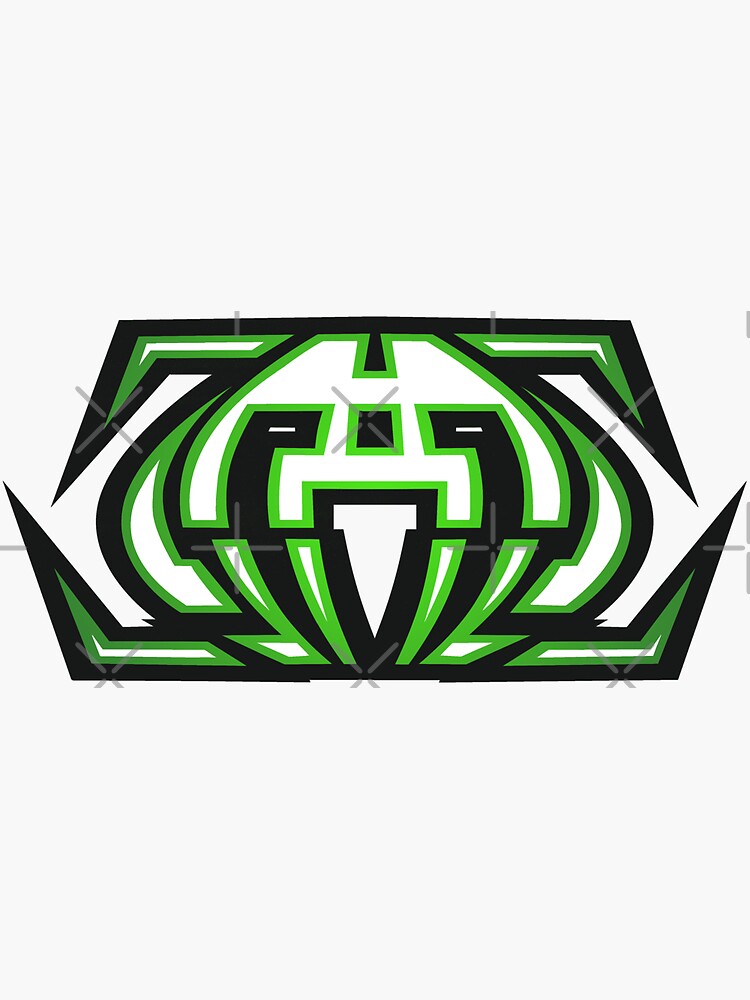The image features a horizontally oriented design on a very light gray, almost beige background. At the core, it showcases an intricate, symmetrical pattern with white shapes forming a central mushroom-like head. This central element includes eye slits with small white rectangles, a form resembling a nose, and a long triangular-shaped white cone at the bottom. Surrounding the central pattern, the design incorporates black and green spiky elements on all sides; the spikes on the top and bottom point inward, creating a complex and dynamic look. The design suggests a symbolic representation, potentially of an animal with horns and fangs, or it could be a stylized tribal logo, possibly for an eSports team or similar. Overlaying the design are faint gray X-shaped watermarks, implying it might be a draft or a protected piece of art. There is no text present on the image.